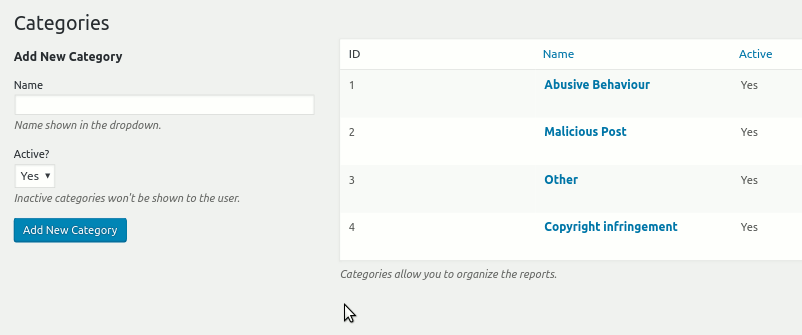The image depicts the "Settings" section of a website or application, specifically designed for managing categories. The background is a light gray color. 

On the left side at the top, bold black letters label the section as "Categories." Directly below, another bold label reads "Add New Category." The interface then presents a field labeled "Name," accompanied by a white, empty textbox. Below the textbox, explanatory text notes, "Name shown in the drop-down." 

Further down, the term "Active" appears, associated with a drop-down box that is currently set to "Yes." An explanation below clarifies, "Inactive categories won't be shown to the user." At the bottom of this section is a button labeled "Add New Category."

On the right side of the image, the columns are labeled "ID," "Name," and "Active." Listed under the "ID" column are numbers one through four. The "Name" column contains the following entries: "Abusive Behavior," "Malicious Post," "Other," and "Copyright Infringement." Correspondingly, the "Active" column indicates that all these categories—"Abusive Behavior," "Malicious Post," "Other," and "Copyright Infringement"—are marked as active.